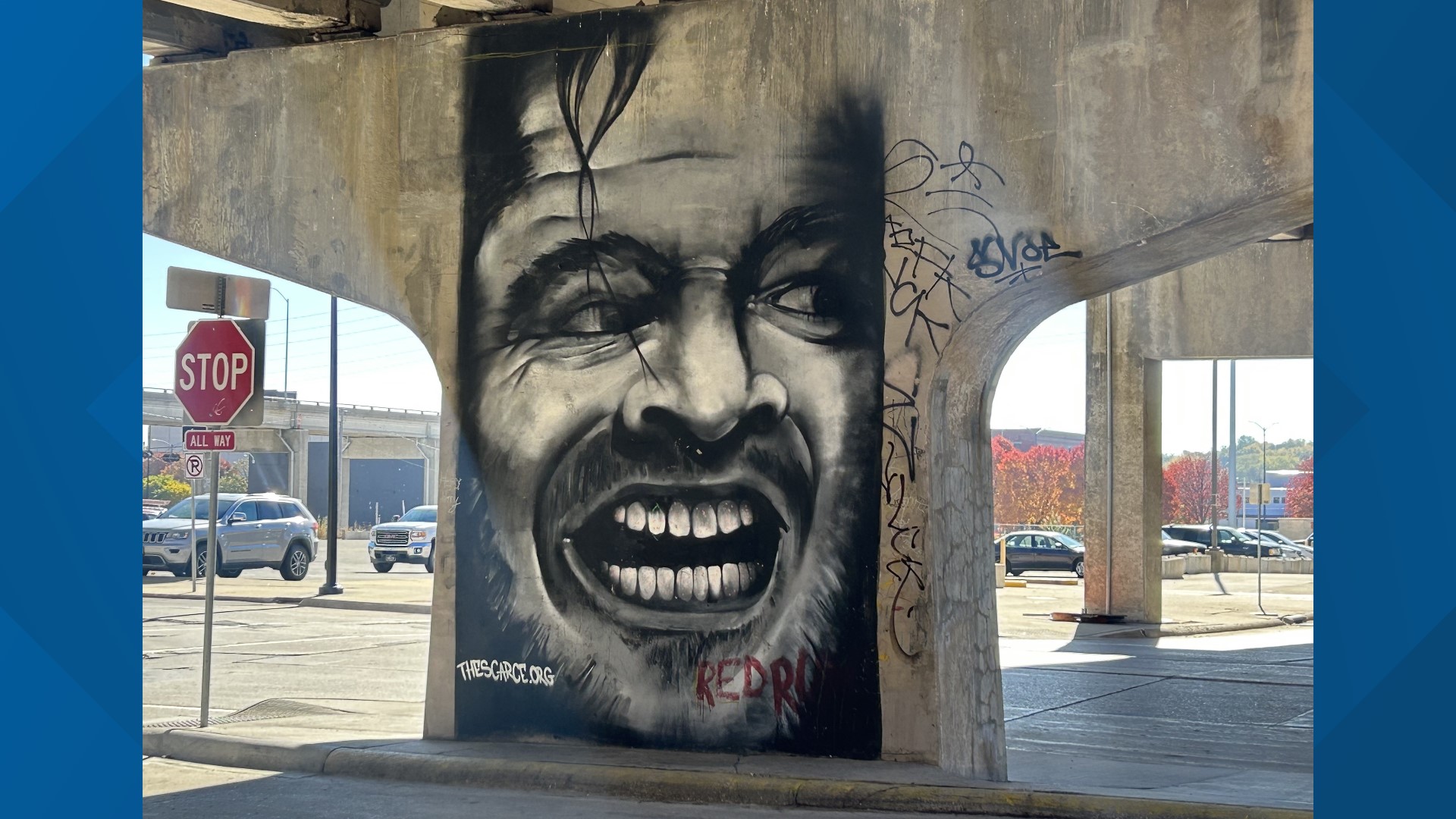The image depicts the underside of a bridge with various features capturing urban and artistic elements. Standing prominently in the center is a large, square support pillar adorned with a striking piece of graffiti. The graffiti portrays Jack Nicholson from the movie "The Shining," his face contorted into a deranged scream, eyes dark and nostrils flared, with disheveled black hair and a scraggly mustache and beard. The artwork, primarily in black and white, emphasizes Nicholson's wide-open mouth and flared nostrils, capturing his intense expression. Below the image, "Red Row" and "Red Rum" are inscribed in red, with another less legible white script on the bottom left, possibly a signature.

Surrounding the graffiti, the under-bridge area teems with urban life. To the left, cars including a silver jeep and possibly a truck, are parked, with a building displaying blue square windows in the background. A prominent stop sign is close to the foreground, indicating an all-way stop. To the right, more parked cars, including a black sedan and a black jeep, align with a scene featuring trees adorned with red and orange autumnal leaves. The bridge itself, a typical stone-gray structure, adds to the gritty urban atmosphere, while a light post stands nearby under the daylight sky. The scene merges the urban environment with a striking piece of pop culture art, creating a visually engaging snapshot.